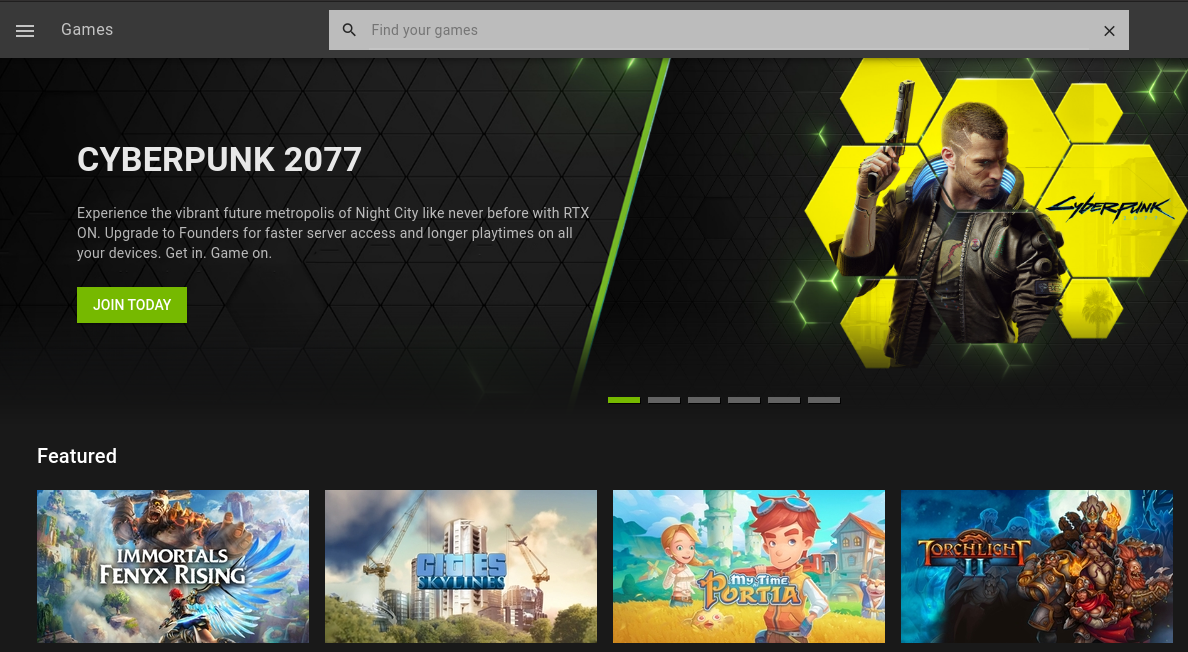The image depicts the interface of a video game launcher from a gaming company. The upper section of the launcher features a light gray bar with the word "Games" positioned on the upper left, accompanied by a three-horizontal-bar menu icon. Adjacent to this is a prominent search bar, labeled "Find your games" in light gray text.

Beneath the search bar, there is a highlighted section for the game "Cyberpunk 2077." On the left, a green button labeled "Join Today" invites users to engage. Between this button and the game's title, a promotional text reads: "Experience the vibrant future metropolis of Night City like never before with RTX on. Upgrade to Founders for faster server access and longer play times on all your devices. Get in, game on."

To the right, the eye is drawn to a vivid image representing "Cyberpunk 2077," adding a dynamic visual element to the launcher. This detailed presentation exudes a sense of advanced technology and immersive gaming experiences.